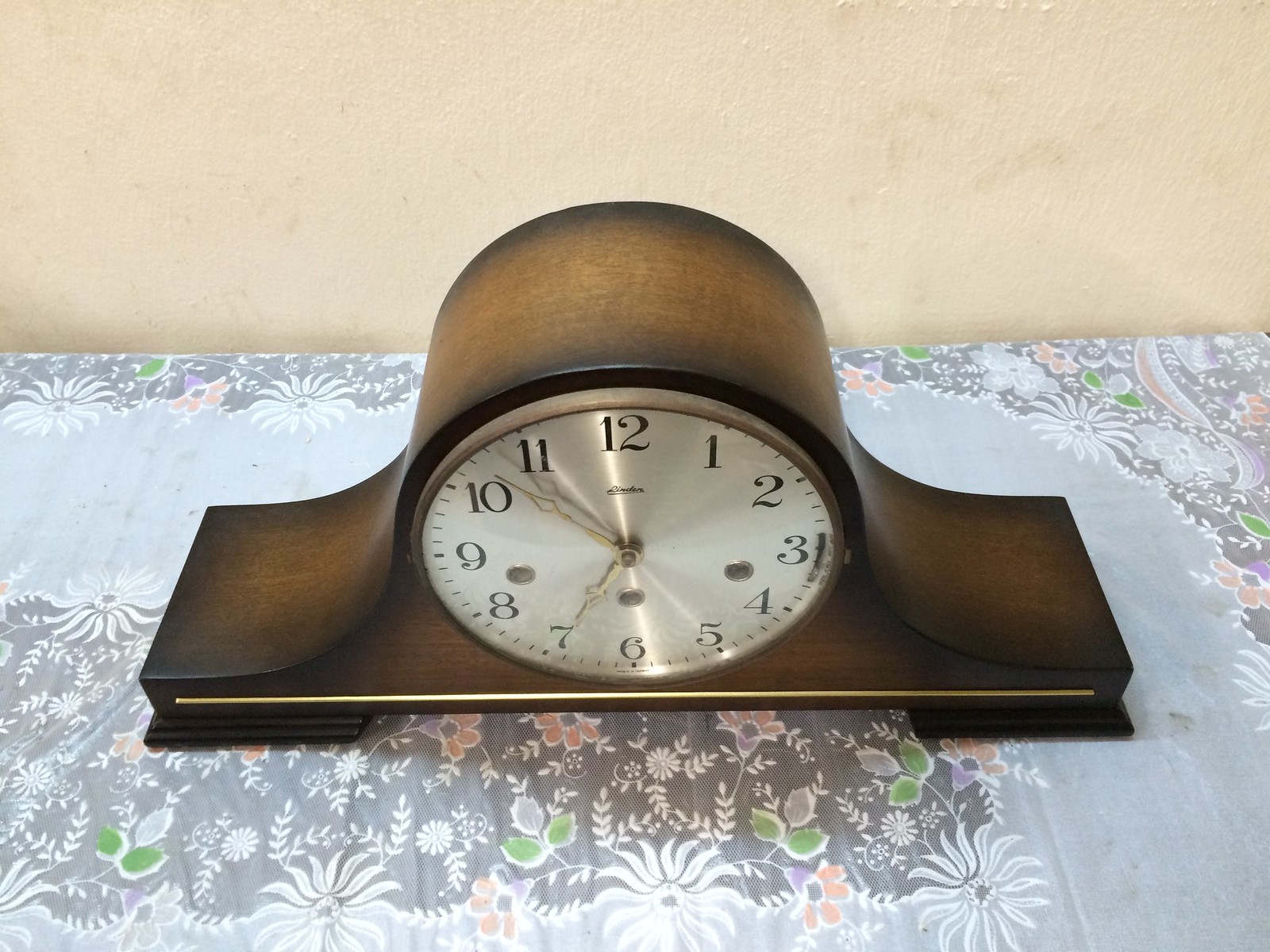This photograph captures an elegantly designed mantelpiece clock placed on a countertop adorned with a floral tablecloth. The clock, with its unique shape, features a smooth wooden frame that curves up into a soft U, lighter in the center and darker around the edges. Its face is a pearlescent white, displaying black numbers from 1 to 12 and thin, metallic gold hands showing the time as 7:52. The tablecloth beneath it is primarily white, decorated with an array of flowers—purple buds, sprouted white blossoms, and orange flowers, accompanied by green and white leaves. The background wall appears to be a light cream color, adding to the serene and elegant ambiance of the scene.